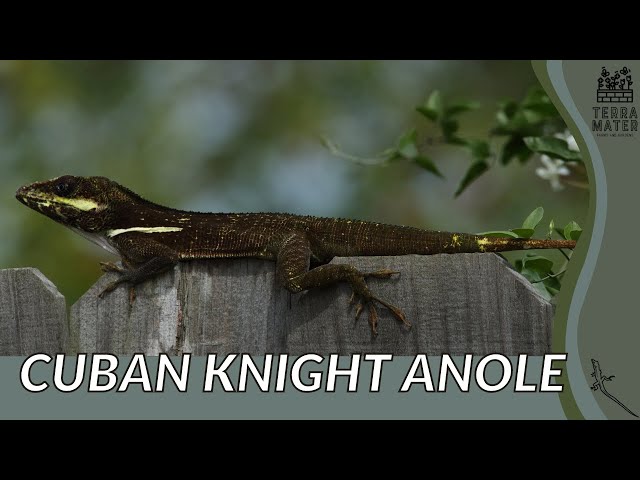The image showcases a Cuban Knight Anole, as indicated by the white caption at the bottom. The photograph is in landscape orientation, capturing the reptile in a striking profile view, facing the left. The anole's skin is a deep brown adorned with distinctive yellow markings; a vertical yellow streak is prominently visible above its front arm, and another yellow streak accents the side of its head. The creature's front and back legs are bent, displaying its slender, toe-like appendages. Its long tail extends gracefully behind it. The anole balances skillfully atop a fence post, adding to the visual intrigue of the scene. In the background, blurred green shapes create a natural, out-of-focus setting, while a green plant is discernible on the right-hand side of the image. The detailed depiction emphasizes the anole's unique coloration and poised stance, set against a subtly vibrant backdrop.